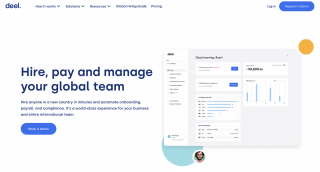The website features a predominantly white background. In the top left corner, there's a small, blue text logo that appears to read "Deel." The navigation menu houses five tabs, with three of them including drop-down options. On the top right, there's a login option next to an indistinct blue bubble.

The main body of the website presents a prominent blue headline stating, "Hire, pay, and manage your global team." Below this headline is a line of small blue text, which is difficult to read.

The main section is divided into two parts: a white column on the left side, which seems to contain some charts and graphs that are too blurry to decipher, and a gray-shaded square on the right. Within the gray square, in the bottom-left corner, there's a turquoise circle with a smaller circle on its right side, featuring an image of a male figure.